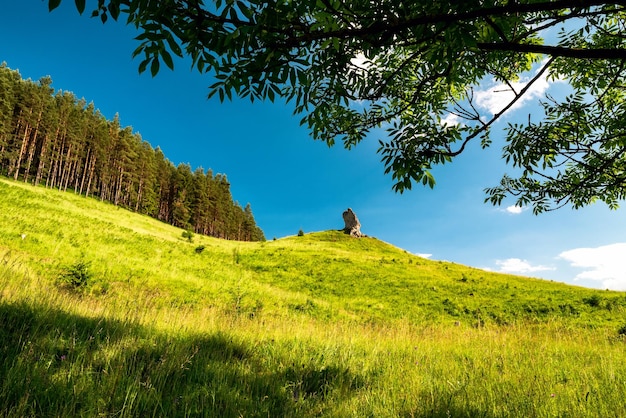The image is a stunning, horizontally oriented outdoor photograph capturing a steep hillside, covered in young, yellowish-green grass that suggests vibrant new growth. From a low-angle perspective, the eye is drawn up the slope towards a noticeable rise, where a distinctive tree stump or similar feature punctuates the landscape. Along the left side of the hill, a row of tall evergreen trees with rich brown trunks and lush green foliage stands prominently. In the background, the brilliant, rich blue sky dotted with white clouds provides a striking contrast to the earthy tones. In the upper right-hand corner, branches and leaves from an overhanging tree partially obscure the view of the sky, adding a layer of natural framing to the scene. The sunlight casts varied shades of green across the valley, highlighting the texture and depth of the grass and trees, creating a captivating and serene visual experience.